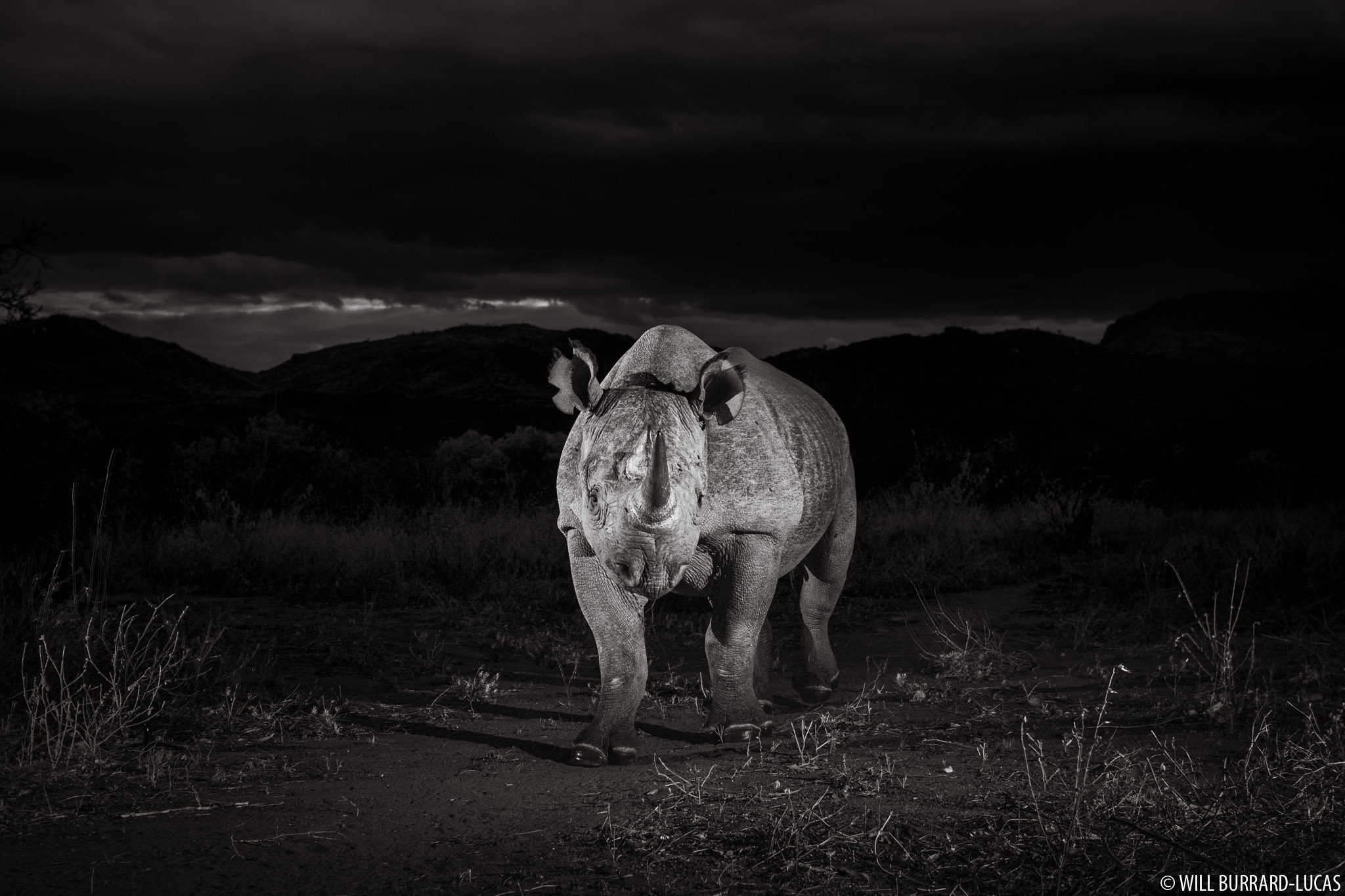This incredible black-and-white photograph captures a rhinoceros in a dramatic nighttime scene, with the atmosphere suggesting either nighttime or very late dusk. The rhinoceros, with its tough grey skin and prominent horn pointed directly at the camera, dominates the center of the image. It stands on a dirt path with sparse patches of vegetation and a bare-earthed surface. The detailed post-processing work adds a touch of surrealism, making the photo appear almost digitally produced. A significant light source illuminates the animal, casting a long shadow across the darkened landscape. In the background, faint outlines of low, vegetated hills and heavy, dark clouds in the sky add depth and mood. The rhinoceros's upright ears give an impression of alertness as it looks straight at the lens. In the bottom right corner, the photo is credited to Will Burrard Lucas, indicating the skilled hand behind this professional work.